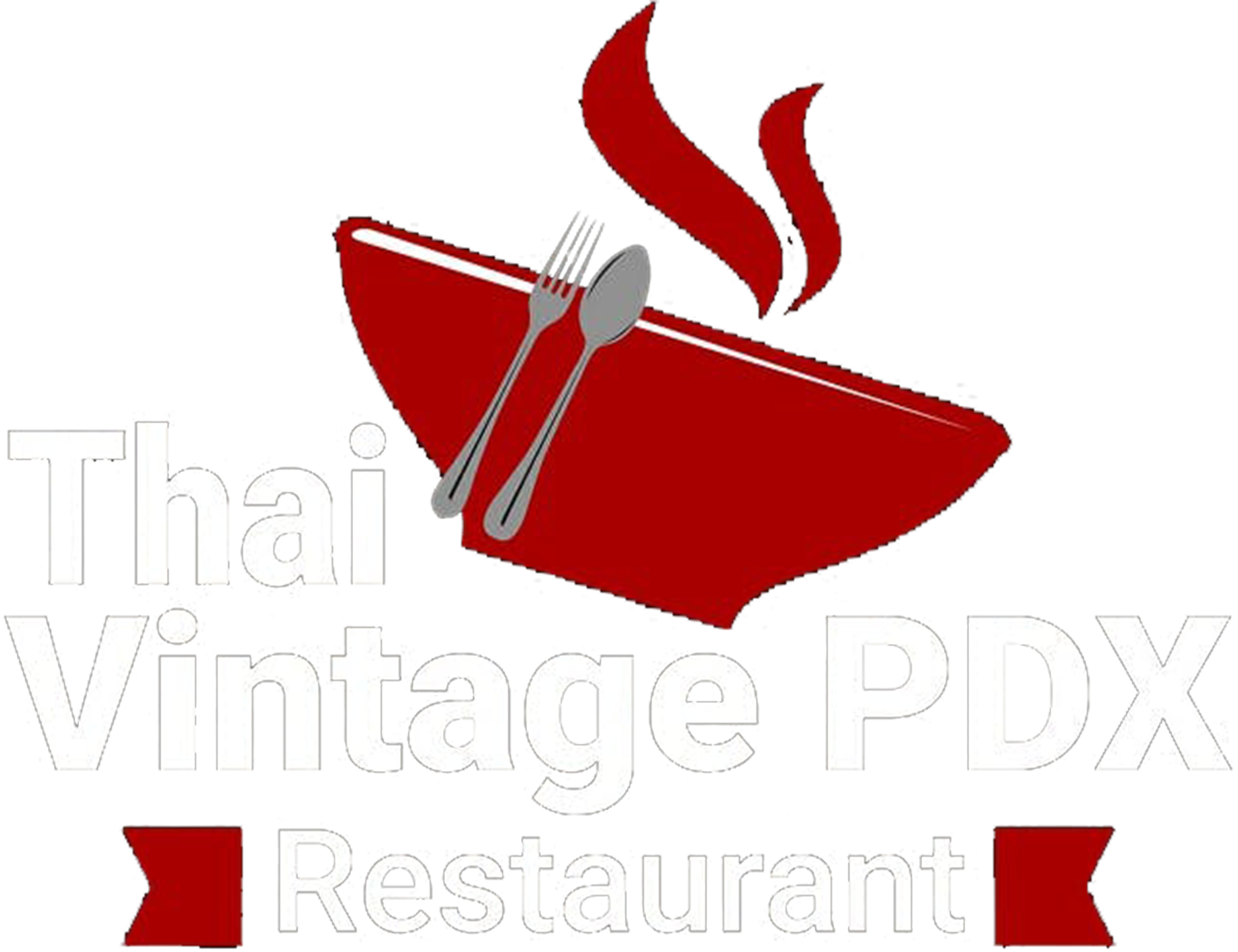The image depicts the logo of Thai Vintage PDX restaurant, featuring a simplistic and roughly-drawn design. Dominating the top center of the logo is a slightly tilted red bowl, crowned with two curved lines emulating steam wafting gently upwards. Nestled within the bowl are a silver fork and a spoon, standing upright, adding to the minimalist charm. Below this imagery, bold white block letters, outlined in black, spell out “Thai Vintage PDX Restaurant.” Flanking this text on either side are red arrow-shaped banners with jagged, uneven lines, pointing inward towards the center. The entire design exudes a hand-drawn, self-made graphic art style that marries crude lines with a sense of vintage authenticity.